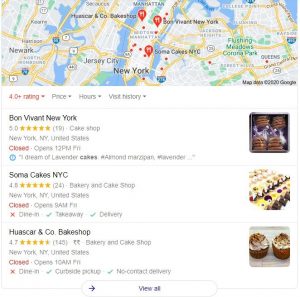This image is a screenshot from Google Maps, showcasing locations in New York with a focus on bakery and cake shop listings. The top part of the image displays a map highlighting areas like New York and Jersey City. Several pins are placed on the map, likely indicating various restaurants.

In the lower right corner, there is a section featuring three specific bakeries. Each listing includes the bakery's name, star rating, review count, service options, and opening hours:

1. **Bon Vivant New York**: Rated 5 stars, this establishment is categorized as a Cake Shop. The status shows it is currently closed, with reopening scheduled for 12 p.m. on Friday. The description reads, "I dream of lavender cakes," along with hashtags #almondmarzipan and #lavender. To the right of this text is an image of cakes.

2. **Soma Cakes, NYC**: This bakery has a rating of 4.0+ stars with 24 reviews. It is also labeled as a bakery and cake shop. Similar to the previous listing, it is marked as closed and will reopen at 8 a.m. on Friday. Service options include take away and delivery. There is a picture of an assortment of cakes next to the listing.

3. **Waskar and Co. Bake Shop**: With a rating of 4.7 stars from 145 reviews, this shop is also a bakery and cake shop. It is currently closed and will reopen at 10 a.m. on Friday. Available services include curbside pickup and no-contact delivery. An oval button beneath the listing reads, "View All," accompanied by a right-pointing arrow.

Overall, the image provides a detailed overview of bakery options in New York City, emphasizing ratings, service availability, and images of their offerings.